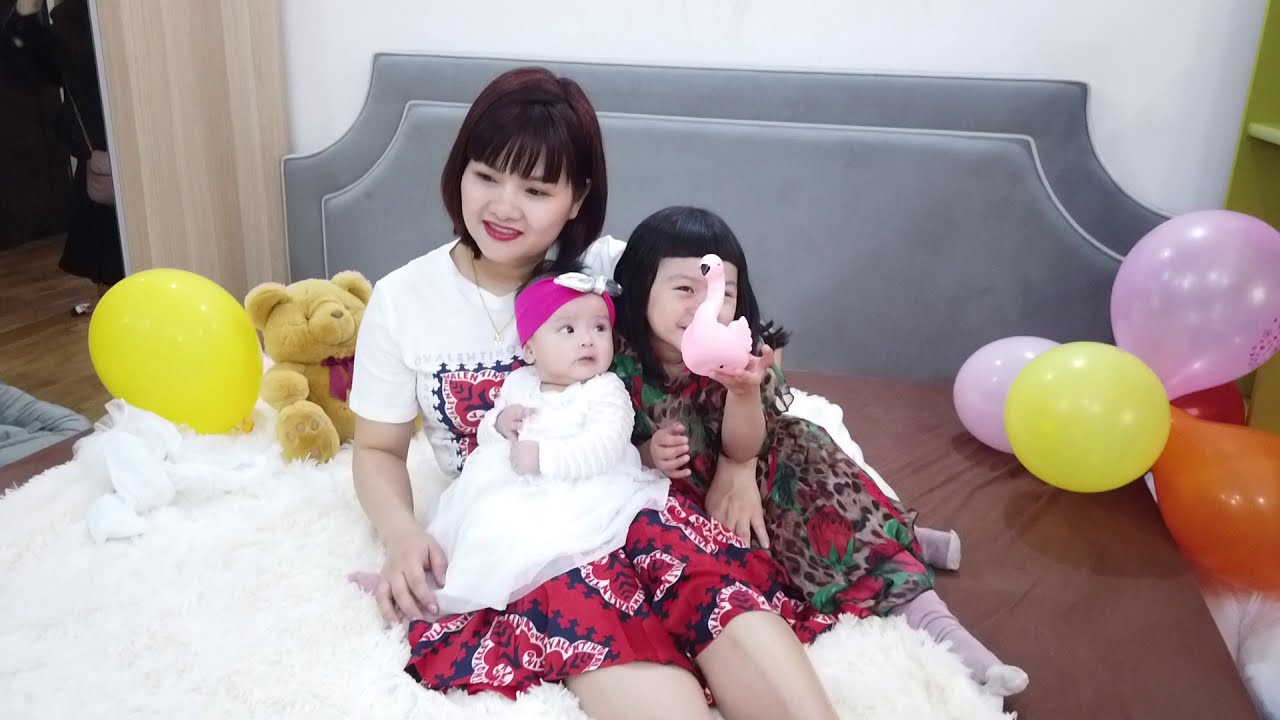This photograph features an indoor setting with three individuals—a mother and her two daughters—sitting on a bed. The mother, who has an Asian complexion, is wearing a white t-shirt and a red skirt, with her baby, dressed in white clothes and a pink headband, sitting on her lap. The older daughter, approximately five years old and wearing a colorful dress, is seated beside the mother, holding a small pink stuffed duck. There is a yellow stuffed teddy bear positioned behind them, and numerous colorful balloons (including yellow, pink, and orange) spread across the bed and room. The room has white walls, and the bed is adorned with a green headboard, a white bedspread over a brown sheet, creating a cozy and vibrant atmosphere. The overall arrangement, with a gray and tan backdrop and abundant decorations, suggests that this might be a professionally arranged photo shoot celebrating family and childhood.